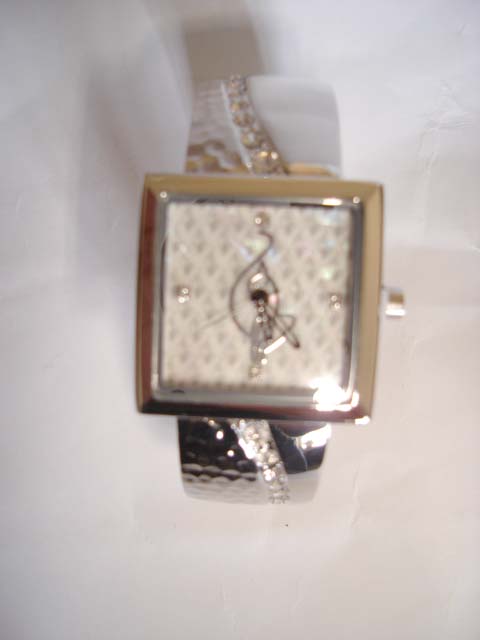This photograph captures an elegant woman's watch from an aerial perspective. The watch face is slightly out of focus, lending a soft blur to the image. The timepiece features a sleek silver square frame, with minimalist markers indicated by silver dots at the 12, 3, 6, and 9 o'clock positions. The absence of numbers adds to its modern design. The background of the watch face showcases a subtle white and silvery diamond pattern, providing a refined contrast to the thin black hands. The band is also silver, embellished with a curved row of glistening diamonds on either side, extending from the watch face. A small, smooth, round silver dial is positioned on the right side of the watch. The entire watch is set against a plain white background, emphasizing its sophisticated details.